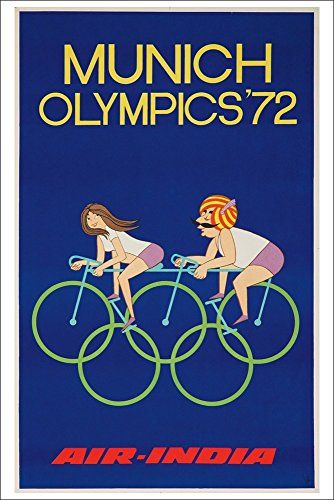The advertisement poster for Air India promoting the Munich Olympics 1972 features a vibrant, eye-catching design. The poster is bordered by a thin black line, followed by a thicker white line, and finally a thin silver line framing the main content. The background of the poster transitions from dark blue at the top to a slightly lighter blue, creating a gradient effect. 

At the top, in bold red and yellow letters, the text reads "Munich Olympics 72". The centerpiece of the poster is a colorful cartoon illustration of a tandem bike with five green wheels, symbolizing the Olympic rings. The bike has a blue frame and seats a woman and a man. The woman, positioned at the front, is depicted with flowing brown hair and wearing pink biker shorts. Behind her, the man sports a distinctive orange and red turban and a thick black mustache, also dressed in biker shorts. Both individuals are illustrated with beige skin tones.

At the bottom of the poster, the text "Air-India" is prominently displayed in red letters. The overall composition is lively and vivid, capturing the spirit of the Olympics and the promotional message of Air India through its engaging and detailed artwork.